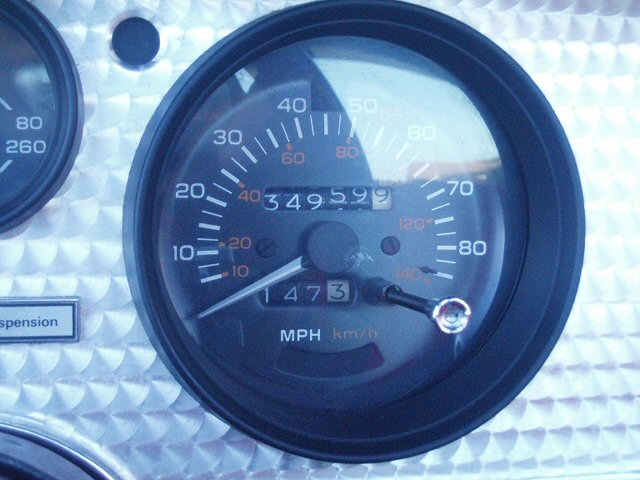The image depicts a detailed view of a car's dashboard, focusing primarily on the instrumentation cluster. On the left side of the dashboard is the main speedometer, which features two concentric bars for speed measurement. The outer bar, marked in white, indicates speed in miles per hour, while the inner bar, marked with orange text, shows speed in kilometers per hour. The speed readings on the outer bar increase in increments of 10 miles per hour, with larger ticks at 10 and 15 miles per hour intervals.

To the right of the speedometer is a knob, likely used to reset the speedometer. Below the speedometer, there is a horizontal meter that currently displays no information. Adjacent to this meter is a label that appears to read "suspension," although only part of the word is visible.

Above the horizontal meter is another gauge, which displays the numbers 80 with slanted marks and 260 with slanted marks to the lower left. There is also a circular opening above this gauge.

The central part of the speedometer has additional markings, showing mileages ranging from 349 to 599, with the number 599 being more prominently displayed. At the bottom of the speedometer, there are numbers "1, 4, 7, 3" positioned next to the reset knob, with a marking of zero as well. The speedometer is covered by circular glass, which has a noticeable glare in the top-right corner.